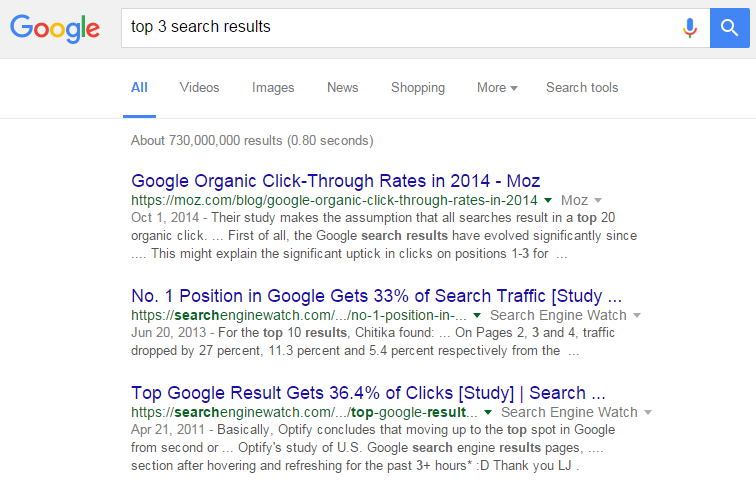The image depicts a Google search results page. At the very top, there's a light gray toolbar with the Google logo in its signature colors on the top left. Below the toolbar, there is a blank search box labeled "top three search results," with a microphone icon to its right. Beside this is a small blue search button featuring a magnifying glass symbol.

Directly beneath the search box are several clickable tabs for different search categories, including "All," which is highlighted in blue with an underline, as well as "Videos," "Images," "News," "Shopping," and a "More" option indicated by a down caret. Further to the right, there is an option labeled "Search tools."

A light gray line separates these tabs from the search results area. Above the results, it displays in light gray text: "About 730 million results (0.8 seconds)." Below this are the top three search results.

Each search result consists of a main title in dark blue, the website URL in green, and a description in black text. The primary search result provides data on Google Organic Click-Through Rates (CTR) from 2014, stating, "Number one position in Google gets 33% of search traffic." The description continues with "Top Google results get 36.4% of clicks. Study [in brackets] search..." There are clickable links for each of the top search results, with URLs provided beneath each title in green text.